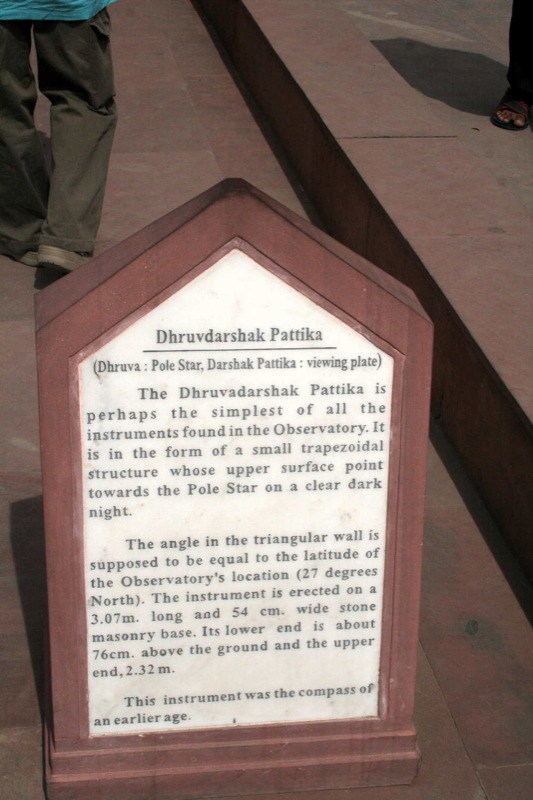The image depicts an informative plaque describing an ancient compass instrument at an observatory. The plaque, resembling both a gravestone and a wooden pentagon, sits atop a reddish, marble-like tiled floor. Made to inform visitors, the plaque reads "Druva Darshak Patika" followed by "Dhruva: Polestar Darshak Patika (viewing plate)." The text explains that this instrument, a small trapezoidal structure, points towards the Polestar on clear nights and is thought to have been the simplest tool in its observatory. It specifies that the angle of the triangular wall aligns with the observatory’s latitude of 27 degrees north and notes the dimensions of its stone masonry base: 3.07 meters long and 54 cm wide, with a height ranging from 76 cm at the lower end to 2.32 meters at the upper end. In the upper left corner of the photo, there's a man wearing dark green pants and a blue shirt, with his knees bent and only his lower body visible. In the top right, a shadow is cast, and a fragment of a leg wearing sandals and brown pants can be seen. The base beneath the plaque features a prominent brown streak running from the top-middle to the right-hand side of the image, adding a distinct feature to the tiled floor.